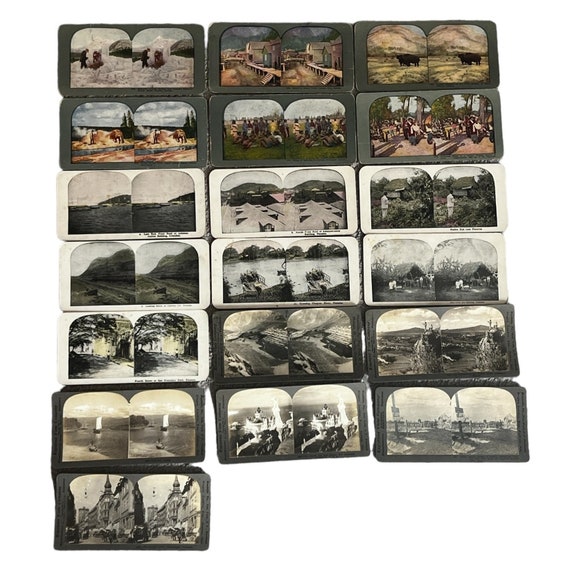This image is a detailed collage of 19 framed photographs arranged in a grid, with three rows and columns, plus one additional image. The photographs are a mix of black-and-white and color, portraying a variety of scenes predominantly focused on historical artifacts and outdoor landscapes. The subjects vary widely, including images of a buffalo, an Indian tribe, a man building an igloo, and a fishing boat. There are also scenes from the Industrial Revolution and New York City, along with cityscapes and nature views featuring animals and greenery. The photographs appear to be both standalone and dual images, possibly comparing before and after scenes. The predominant colors in the pictures are white, green, black, gray, yellow, and red. There is no text accompanying the images, and the overall theme seems to center around Northern American history and significant historical events or daily life from various periods.